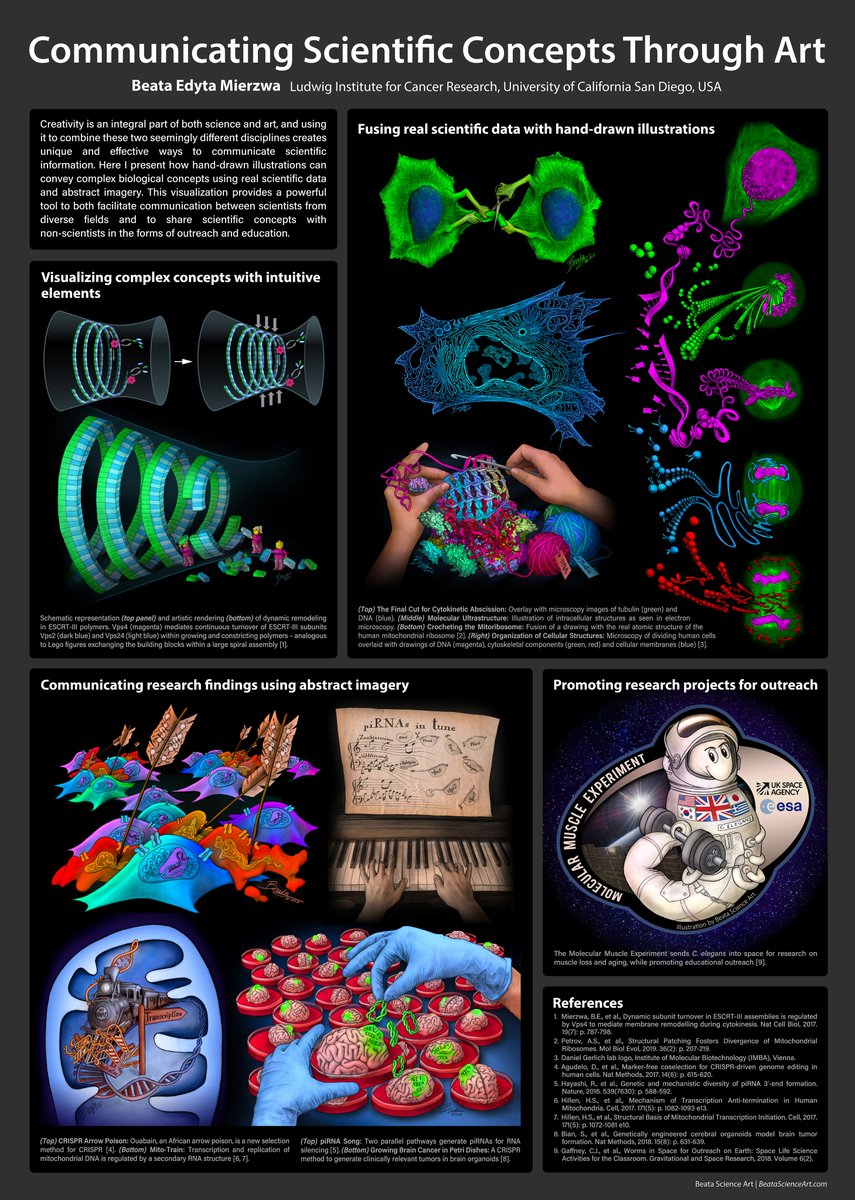The poster, titled "Communicating Scientific Concepts Through Art," spans the entire top section in white text on a dark grey background. Credited to Beata Adita Merza from the Ludwig Institute for Cancer Research, University of California, San Diego, it is structured into several box-like sections, some larger than others. The top left section features small white text, accompanied by diagrams of blue lines on grey backgrounds. Adjacent to this, the top right section showcases a blend of real scientific data with hand-drawn illustrations, depicting structures such as ribosomes and DNA, often in neon colors. 

Below, the left section displays diagrams labeled "Visualizing Complex Concepts with Intuitive Elements," with various scientific illustrations, including hands knitting DNA-like strands. To the right, another section illustrates "Communicating Research Findings Using Abstract Imagery," showing diverse visuals like blue-gloved hands handling brain specimens, piano playing, and stylized sea creatures.

The bottom right corner highlights an amusing depiction titled "Promoting Research Projects for Outreach," featuring a cartoon astronaut adorned with the flags of the United States, South Korea, Great Britain, and Japan. The very last box in the bottom right says "References," listing numerous sources in small white type. Overall, the poster intricately combines scientific concepts with artistic expressions to enhance understanding and engagement.